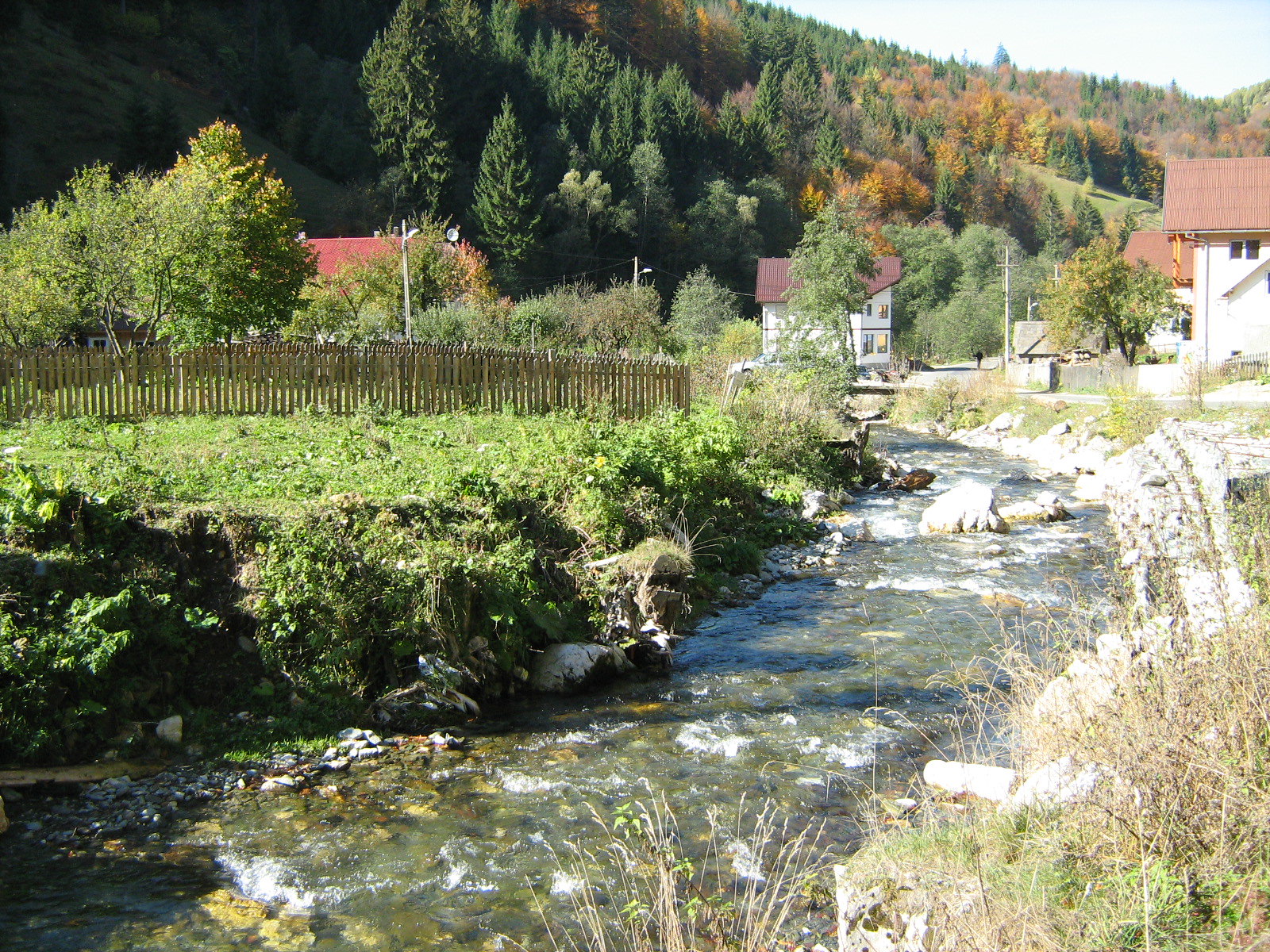This picturesque landscape captures a serene outdoor scene, likely at the foot of a mountainous area resembling the Smoky Mountains. Central to the image is a clear, meandering stream beginning at the lower left, moving up towards the middle right, and curving back towards the left. The stream's bed and surrounding rocks are visible, with a built-up grassy area on the left providing a stark contrast due to its steepness. Beyond this rise, a wooden fence can be seen, alongside trees and bushes, with the red roof of a house peeking through. Further behind the house, a hill adorned with a dense forest of trees in various shades of green and orange signifies the fall season. On the right, the landscape features lower shrubs, some brown from dryness, more rocks, and additional shrubbery. Nestled here are two white, rustic houses, one with a copper roof, adding to the quaint village ambiance. The background further extends to reveal another house, a tree, and a distant hill covered with trees. The light blue sky at the top right adds to the overall tranquility of the scene, making it a beautiful and inviting place to visit, perfect for immersing oneself in nature on a warm summer day.